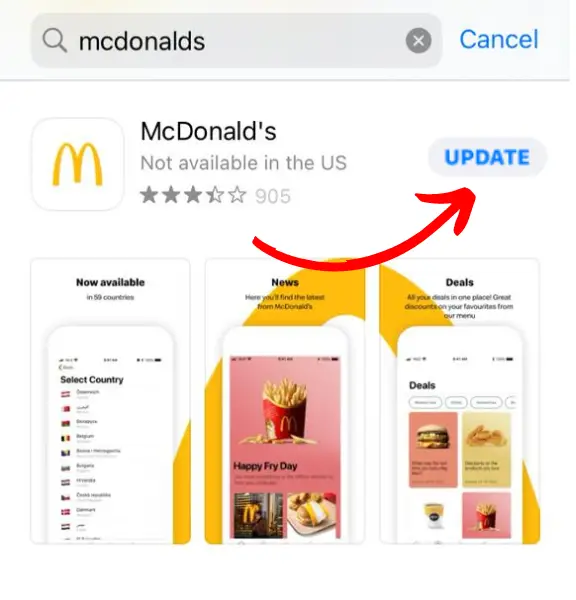The image depicts a close-up view of a search interface for "McDonald's." In the upper left-hand corner, there is a search bar against a gray background. To the right of the search bar, the word "Cancel" appears in blue font with a capital "C." Below this, a gray separator bar extends across the width of the image. There is blank space beneath this separator before the main content begins.

Starting from the left, there is a white square icon featuring a yellow 'M,' the recognizable symbol of McDonald's. To the right of the icon, "McDonald's" is written in black font. Below this, in gray font, it states "Not available in the US." Further down, the rating of "4.25 stars" is displayed along with "905 reviews" in close proximity. To the right of this text, there is an arrow pointing towards the "Update" button, which suggests an update is available for the McDonald's app.